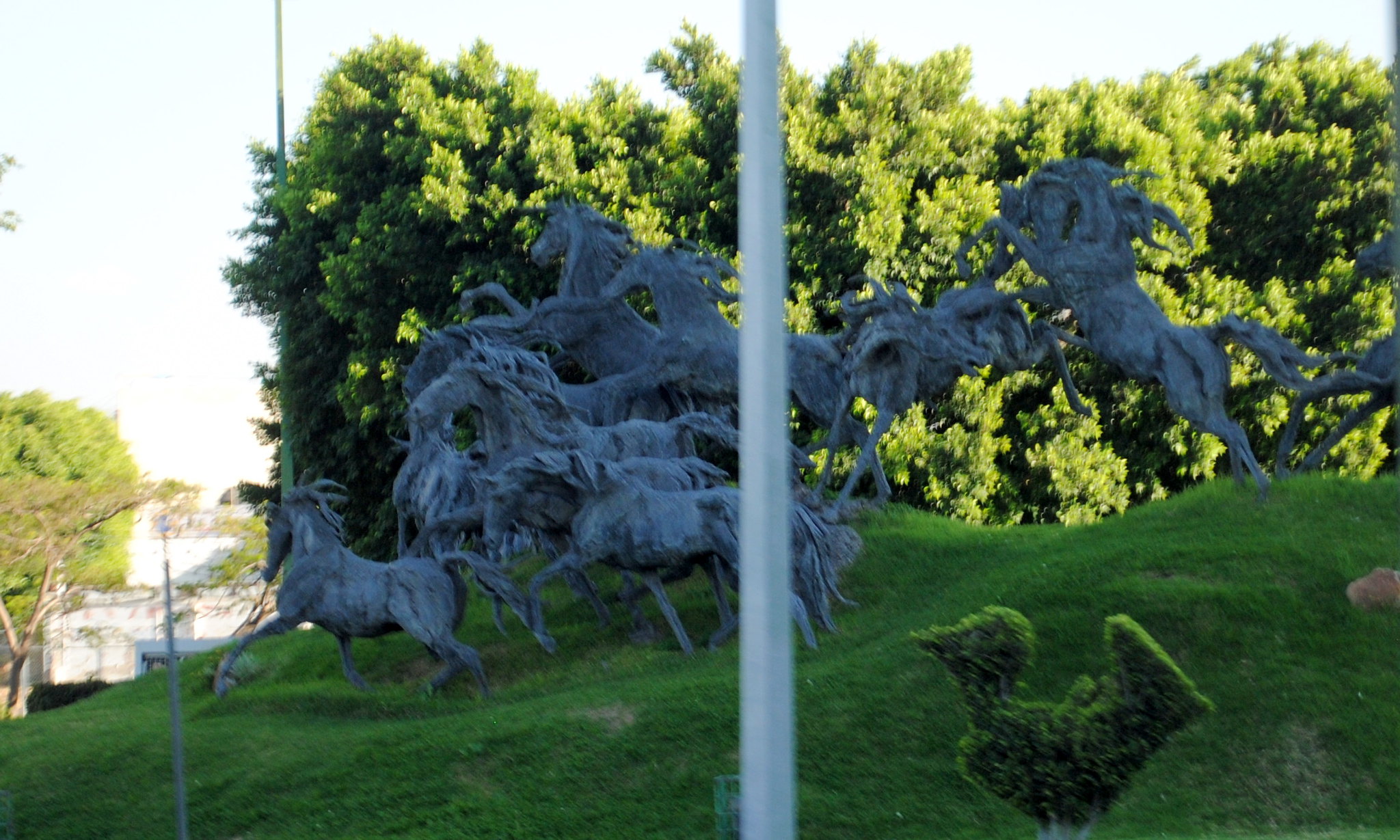In this captivating image, an intricate sculpture featuring a dynamic grouping of wild horses is set amidst a lush, hilly landscape. The horses are captured in various phases of motion; some are galloping on all fours, others are rearing up on their hind legs, and a few appear to be leaping. This lively scene conveys the essence of a stampede through a meticulously manicured green field. The horses themselves are rendered in a bluish-gray hue, and their detailed forms convey a sense of urgent motion and freedom.

The backdrop includes tall, leafy trees in rich green shades, creating a dense foliage barrier that extends to the horizon. Despite the somewhat cloudy sky above, the area is brightly illuminated by sunlight, highlighting the vibrantly green grass and the well-tended shrubs. Off to the side, a neatly trimmed hedge has been sculpted into the shape of a duck, adding a whimsical touch to the natural setting.

There is also a noteworthy element in the form of a slender white pole rising from the ground, whose purpose or top cannot be discerned from the image frame. Additionally, to the left side of the image, behind the undulating hills, one can glimpse the white facade of a building, potentially a house, surrounded by more trees, further adding to the picturesque and serene environment.